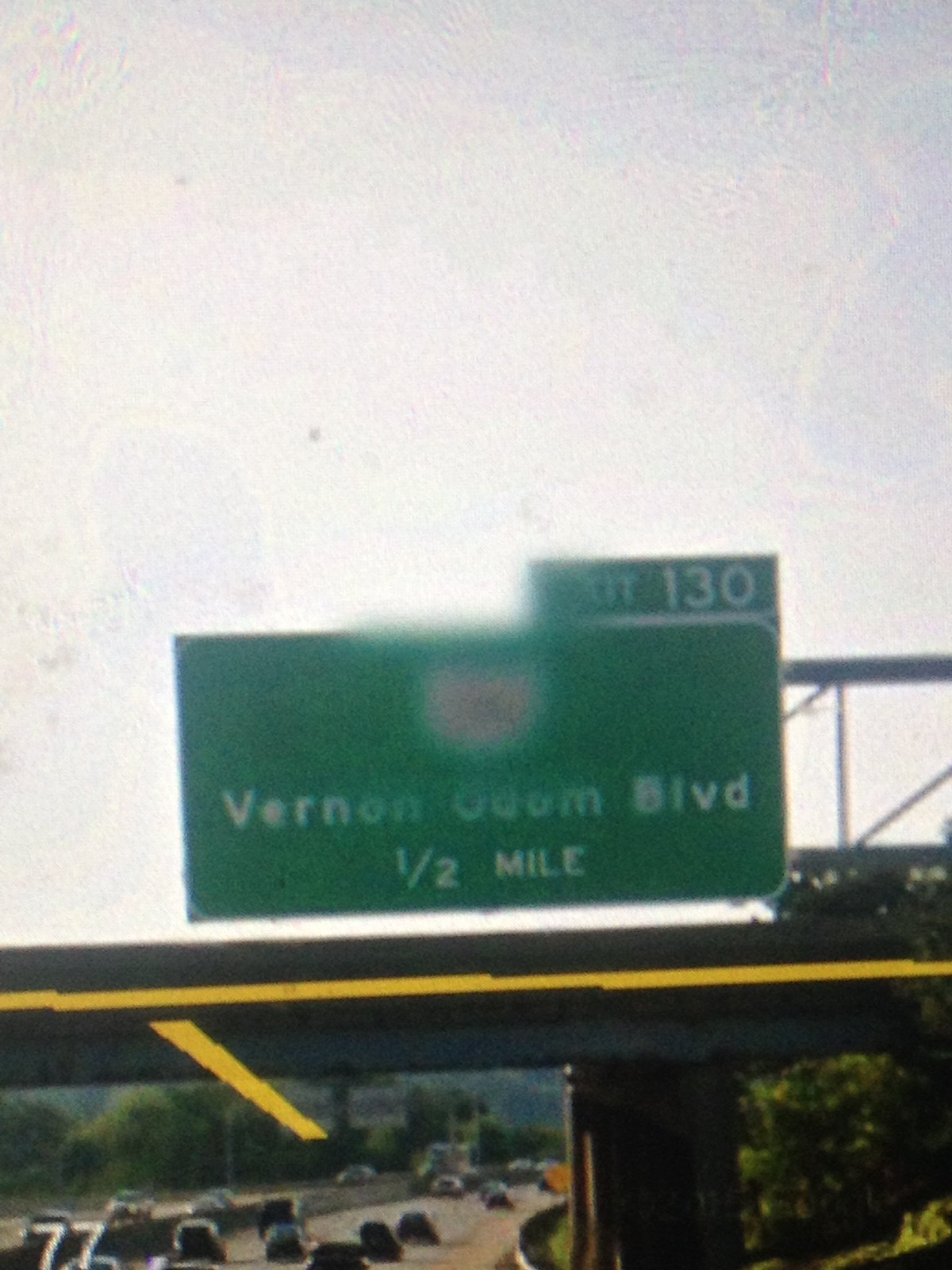This vertically-oriented color photograph captures a blurry scene of a large green exit sign on an interstate highway. The sign, emblazoned with white text, reads "Exit 130" prominently in the top right corner and indicates "Vernon-Odom Boulevard, 1/2 mile" below. The top portion of the image is consumed by a washed-out, cloudy sky. In the background, an overpass spans from left to right, with several cars visible on the freeway below. A prominent yellow line, possibly a reflection or an edited marking, runs diagonally across the image from bottom left to bottom right, with a shorter yellow line beneath it pointing downward. The landscape features trees on the right side of the road and in the distance to the left. Additionally, a yellow diamond-shaped sign is seen near the road, adding to the roadside details.